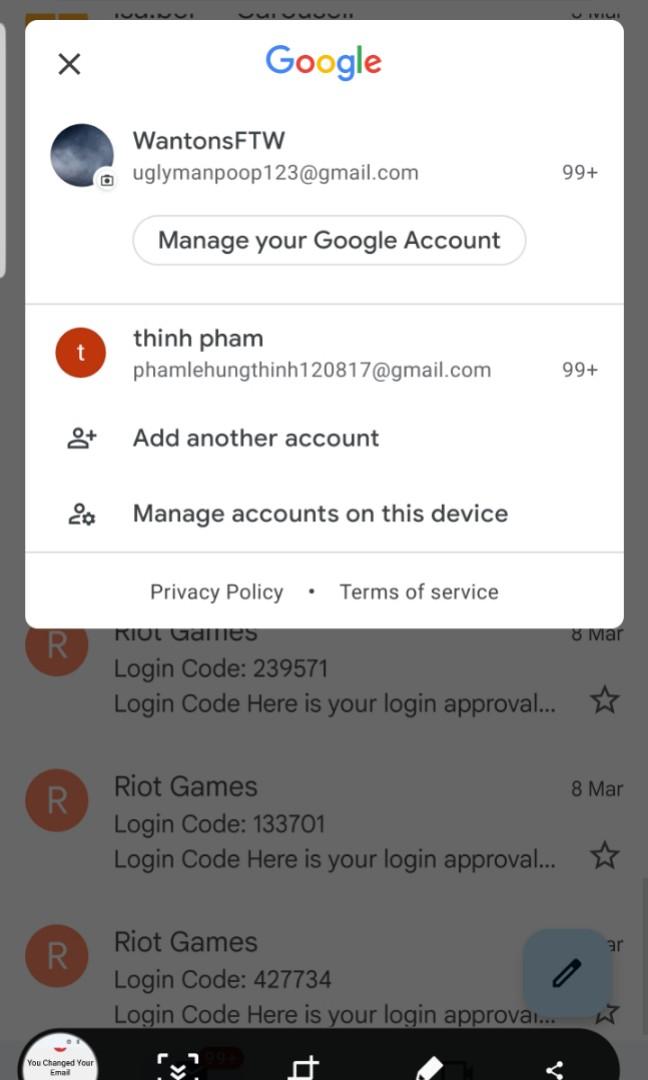This screenshot, taken from a tablet or smartphone, depicts a Google settings pop-up. The pop-up, housed in a white rectangular box, features a black 'X' on the top left, and the Google logo prominently displayed in the center. The Google logo is characterized by its distinct color scheme: a blue 'G,' followed by a red 'O,' an orange 'O,' a lowercase blue 'g,' a lowercase green 'l,' and a lowercase red 'e.'

On the left side, there is a profile picture displaying storm clouds in shades of blue, black, and gray. To the right of the profile picture, it reads "WANTONS FOR THE WIN" in all capital letters. Below this, in gray text, the email address "UGLYMANPOOP123@gmail.com" is displayed, accompanied by a notification indicating "99+" on the right side.

A bold black button labeled "Manage your Google Account" is situated under the email information. Further down, a red circle containing a white 'T' and labeled "THINH PHAM" is visible, showing the email address "PHAMLEHUNGTHINH120817@gmail.com" with another "99+" notification on the right.

Two additional options in bold black text follow: "Add another account" with an accompanying silhouette icon and a 'plus' sign, and "Manage accounts on this device" with a gear icon. Near the bottom, in gray text, it reads "Privacy Policy" and "Terms of Service."

In the background, multiple emails from Riot Games are visible, each containing different login codes: "23957," "133701," and "427734." The screenshot also captures the editing software interface at the bottom of the screen.